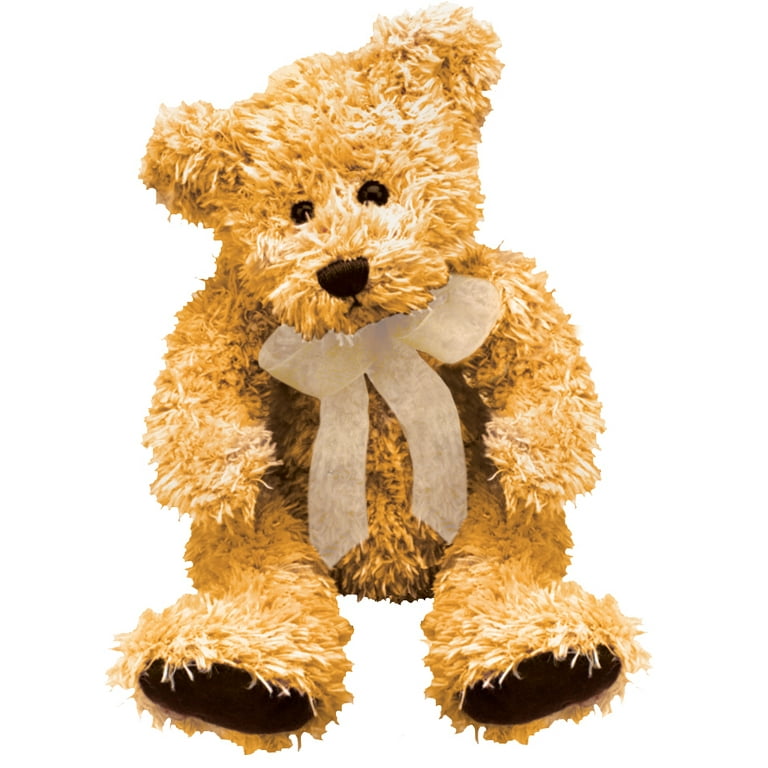This image features a professionally staged and taken photograph of a light brown, very fluffy teddy bear set against a purely white background, reminiscent of a stock photo found in Amazon listings. The teddy bear possesses a cute, cuddly appearance with its soft, fuzzy fur that resembles yarn strings. It has shiny brown button eyes and a button-type dark brown nose, embroidered with black thread to form a small mouth beneath. Around its neck is a sheer white ribbon tied into a bow, through which you can see some of the bear's yarn texture. The bear's feet, positioned closest to the camera, have dark brown soles. The bear's head is slightly tilted to the left, enhancing its charming and endearing look, making it an ideal gift for both children and adults who love cute, plush teddy bears.